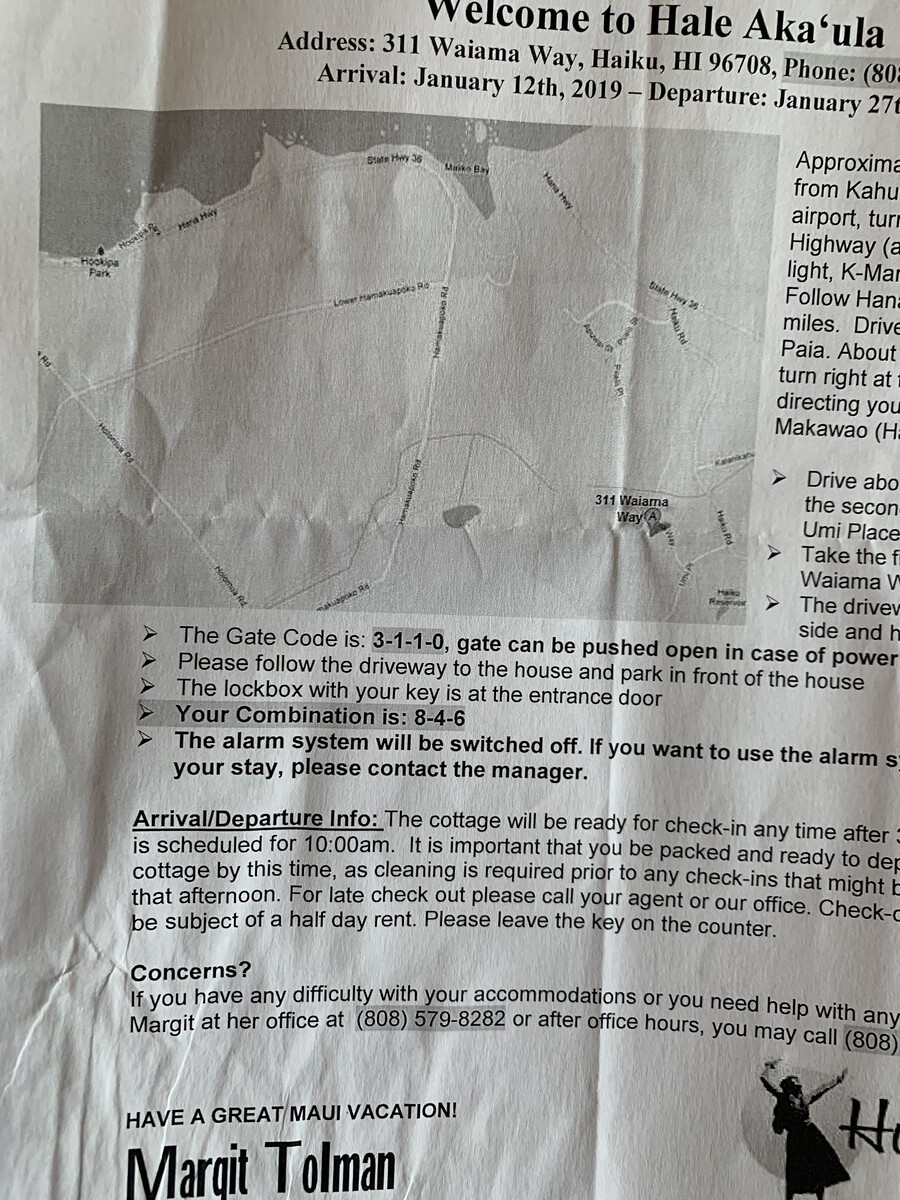The image depicts a badly wrinkled and creased off-white paper print, possibly an informational pamphlet for an accommodation, such as an Airbnb, with several text fragments cut off. At the top, "Welcome to Hale Aka'ula" is printed in bold letters, with the address "311 Wai'ama Way, Haiku, Hawaii, 96708," followed by the dates "Arrival: January 12, 2019" and "Departure: January 27." Next to this text, there is a partially obscured phone number and a gray map of Hawaii. An image of a human figure with an outstretched arm towards the horizon and a large letter "H" are also visible. The document includes various sections with directions and information about arrival and departure, including instructions about gate codes and parking details. Concerns are addressed to a manager, with a contact number "808-579-8282." At the bottom left, the text "Have a great Maui vacation, Margit Tolman" is clearly printed.